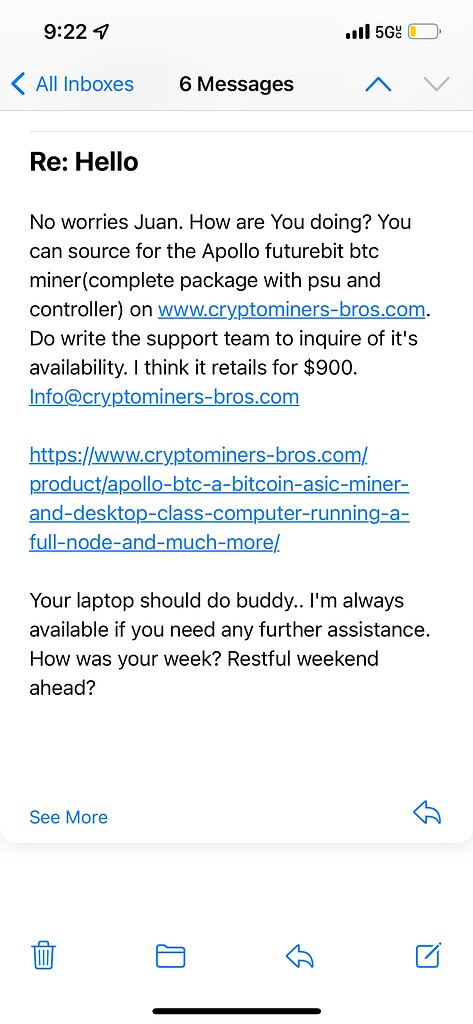This is a detailed screenshot from a person's smartphone. The screen shows the status bar at the top with the time displayed as 9:22. The device has full network coverage with four bars and is connected to 5G. The battery indicator is yellow, suggesting the battery is running low. Below the status bar, there is a blue back arrow icon on the left side of the screen.

The main part of the screenshot displays an email inbox under the title "All Inboxes," indicating that there are six unread messages. The highlighted email subject reads "Re: hello." The email body starts with "No worries Juan. How are you doing?" The email continues with information on sourcing the Apollo FutureBit BTC complete package, including PSU and controller, from www.cryptominers-bros.com. It advises writing to the support team to check its availability and mentions that the package is likely priced around $900. Further, it suggests that the recipient's laptop should suffice for the task and offers personal assistance if needed. The email closes with casual inquiries about the recipient's week and upcoming weekend.

At the bottom of the screenshot, there are four icons: a trash can (for deleting emails), a folder (for organizing emails), a left-pointing arrow (likely for replying to or forwarding the email), and a notepad icon (likely for composing a new email).